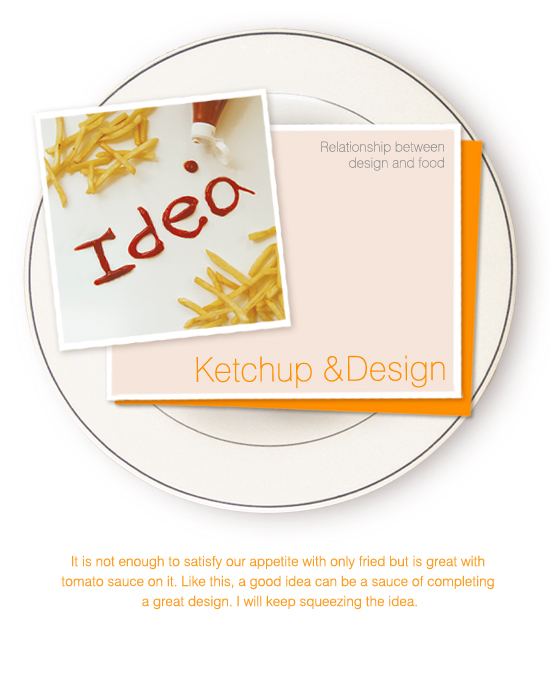This detailed photograph showcases a conceptual composition featuring a white dinner plate with a black rim, set against a white background. On the plate are three overlapping, digitally altered squares: the bottom square is orange, the middle one is light orange with text, and the top one is white. 

On the topmost white square, the word "Idea" is artistically written in ketchup, accompanied by a photo of french fries and a ketchup bottle peeking from the corner. Text along the bottom reads, "It is not enough to satisfy our appetite with only fried, but it is great with tomato sauce on it. Like this, a good idea can be a sauce of completing a great design. I will keep squeezing the idea." 

The middle light orange square bears the phrases "Relationship between design and food" and "Ketchup and design." The composition alludes to the idea that good design, similar to a great meal, can be enhanced and completed with the right "sauce" – in this context, a creative and innovative idea.